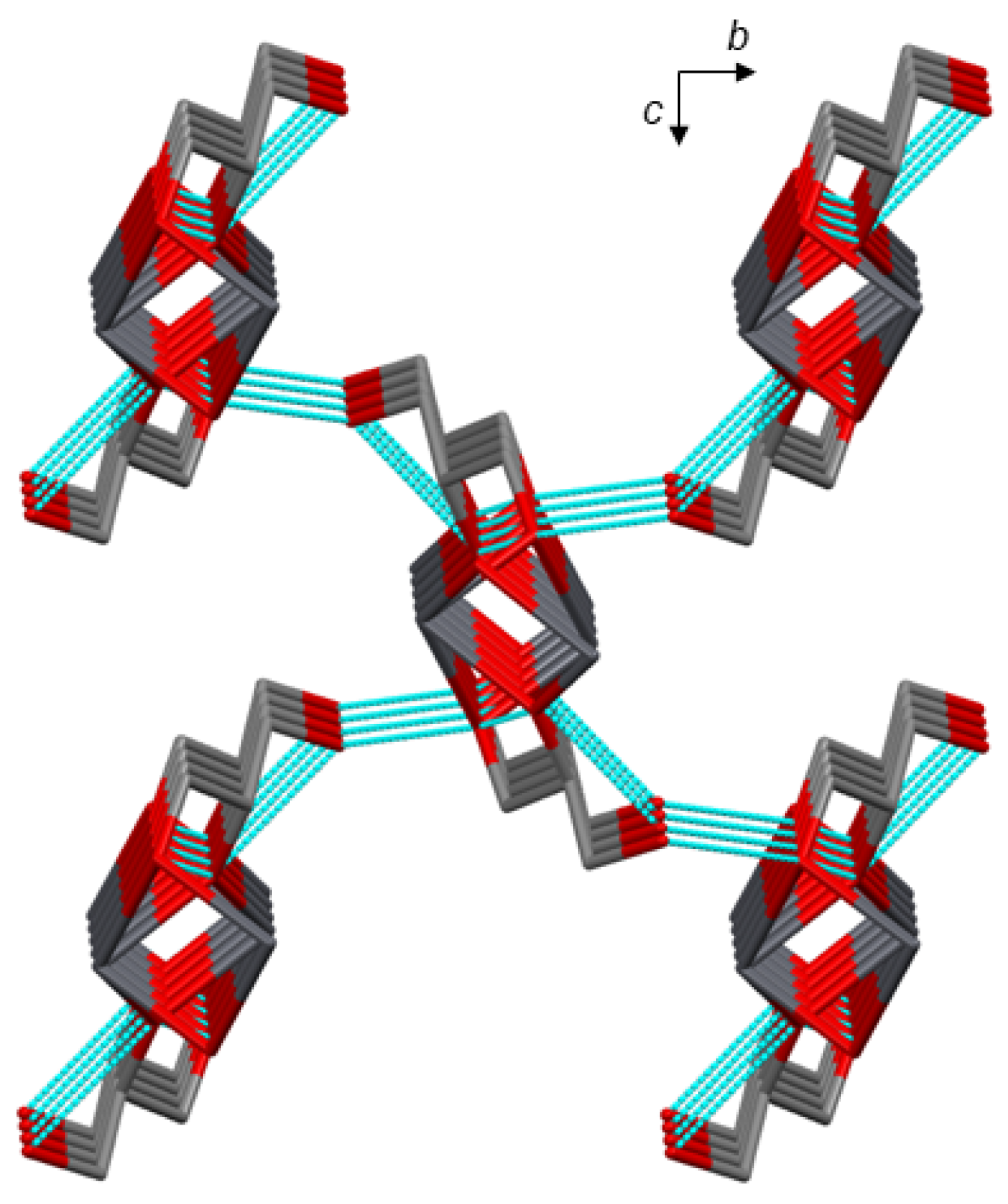The image, resembling an abstract computer-generated design or a textbook diagram, prominently features a right angle formed by two interconnected arrows at the top-right corner. The arrow labeled 'B' points to the right, while the arrow labeled 'C' points downward. The main structure within the image has a mechanical, almost transformer-like appearance, with elements that might be magnets or metal objects showing red tips and gray middles. Interspersed among these are light blue, turquoise-hued segments that look reminiscent of Legos. This central structure extends in four distinct directions—down left, down right, up left, and up right—resembling staggered steps or angular ribbons. The overall design is boxy and intricate, made up of several squares forming a cohesive yet complex pattern, colored in shades of red, turquoise, and gray. The image might be interpreted as a mathematical equation or a DNA strand due to its detailed and systematic layout, but its true purpose or depiction remains abstract.